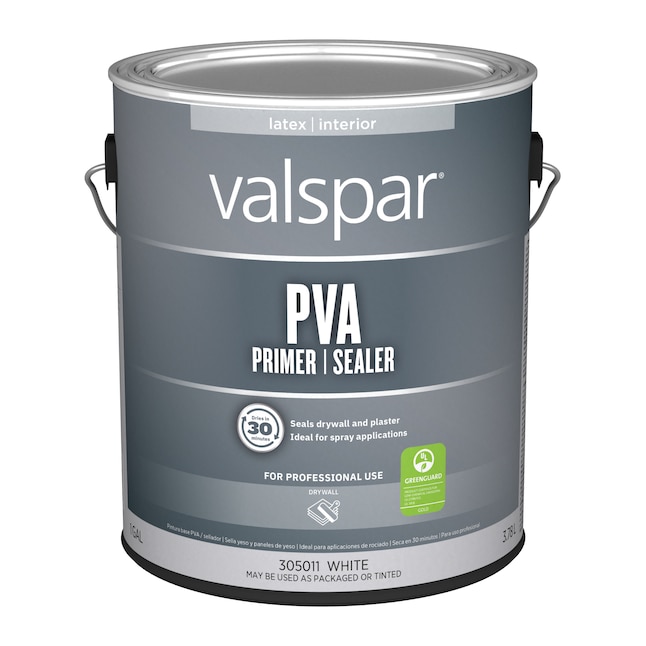This image features a Valspar primer and sealer paint can, predominantly in dark gray with various white and light gray details. The cylindrical can, clearly unopened, sports a thin metal handle visible at the back. The silver lid at the top is securely in place. Just beneath the lid, a light gray strip bears the designation "Latex Interior" in white lettering. The central portion of the can is marked by the Valspar brand name followed by the text "PVA Primer Sealer." Further down, an array of details includes "Seals Drywall & Plaster, Ideal for Spray Applications" in white lettering and a small white emblem with arrows encircling the number "30." A small green sticker toward the bottom suggests environmental friendliness, though the text within the sticker is unclear. The last line of text displays the product code "305011 White" along with a note stating "May Be Used as Packaged or Tinted," all set against a light gray band with black text and a black trim encircling the base.